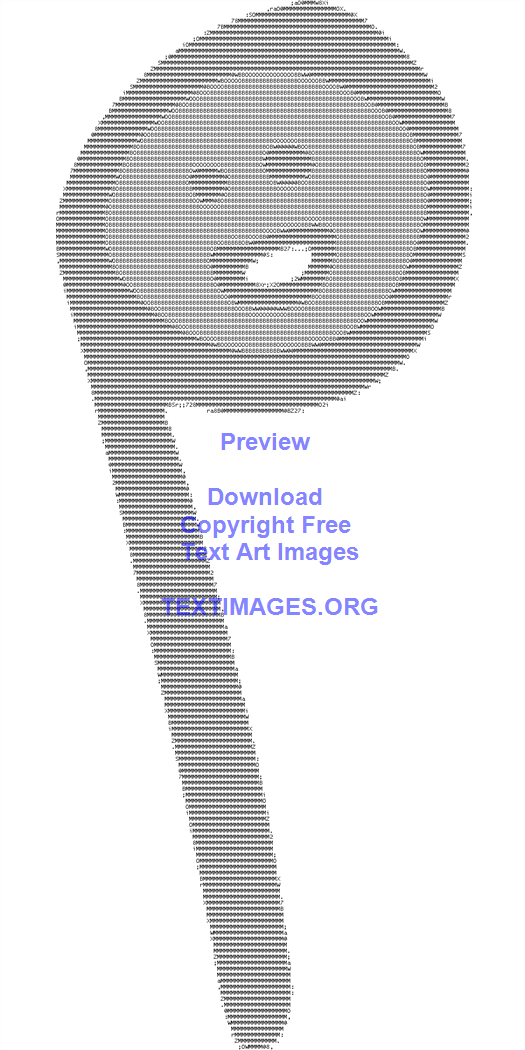The image features a stylized design resembling the letter "P," intricately crafted using various numbers and characters, giving it a text art appearance. At the center of the "P," there's a simplistic face with two eyes and an open mouth, evoking a cartoony expression. The colors in the artwork range from dark gray to light gray, creating a sense of depth and texture, all set against a clean, white background. Accompanying the graphic is a light blue text that reads: "preview, download copyright-free text art images, textimages.org." This unobtrusive yet informative text situates itself below the main design, emphasizing the image's function as an example of downloadable text art available from the mentioned website.